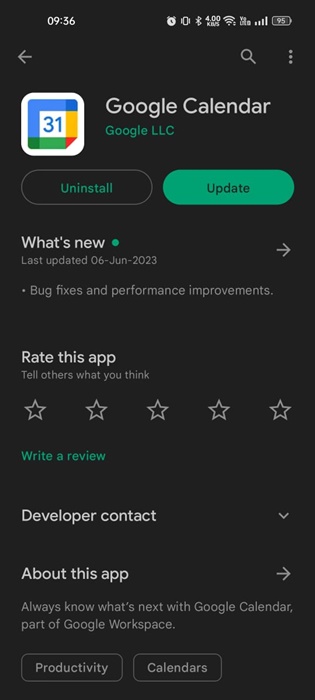A detailed screenshot of a cell phone screen illustrates the process of downloading the Google Calendar application in night mode. The screen background is black, providing a stark contrast to the white text and icons. 

In the top left corner, the current time is displayed as "9:36" in white. Adjacent to this are icons indicating various statuses: an alarm is set, Do Not Disturb mode is activated, Bluetooth is on, and the service and Wi-Fi signals are active. The battery icon shows a 95% charge.

Below these notifications, the navigation buttons for back and search are visible. 

The focal point of the screenshot is the Google Calendar application by Google LLC. Buttons for "Uninstall" and "Update" are prominently displayed: the uninstall button in black with green text, and the update button in green with black text.

A section below outlines recent changes to the app, noting, "What's New: Last updated June 6, 2023," followed by a bullet point indicating "bug fixes and performance improvements."

Further down, users are prompted to rate the app and share their thoughts. There are five selectable stars for rating, with a "Write a review" option highlighted in green text.

The section for "Developer contact" is indicated in white text with a drop-down arrow for additional information. Finally, the "About this app" section provides a detailed description of Google Calendar.